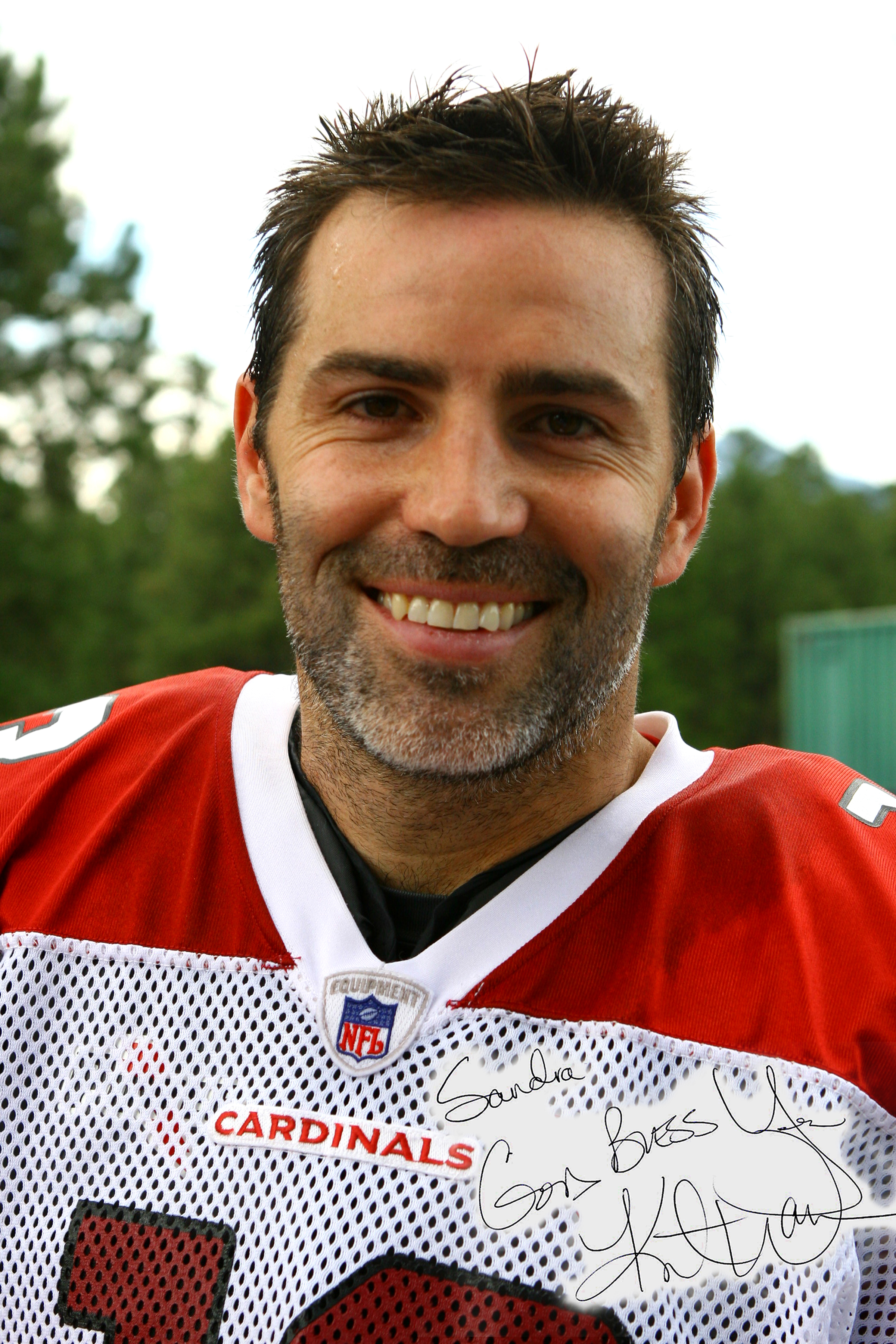This is a detailed headshot photograph of an NFL football player in his late 30s to early 40s. He is smiling and donned in a red and white jersey that bears the team name "Cardinals" in red beneath the neck, along with the "NFL Equipment" logo situated just above that. The red extends from the shoulders down to a white mesh net beneath, designed for breathability. The player has spiky, short brown hair, with a grey, scruffy stubble predominantly greyer around the chin. His dark eyes reflect a sense of warmth. The background is a blur of greenery, possibly trees and bushes, beneath a clear sky. In the bottom right corner, there is a handwritten note that says "Sandra, God bless you," followed by an indistinct signature that appears to read something close to "Caltran."